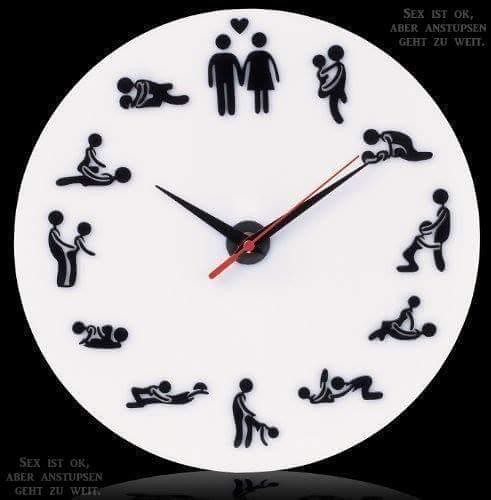The image is a detailed color artwork featuring a unique clock against a black background. The clock's face is a stark white circle with a black border. Traditional numbers are replaced by ideograms of people in various sexual positions. At the 12 o'clock position, a man and a woman are depicted in black and white, identifiable by their stylized figures reminiscent of restroom symbols. They hold hands with a heart symbol above their heads, signifying a symbolic start or end. As the positions advance clockwise, different explicit poses replace the usual numerals. The clock shows a time of 10:10, marked by three hands: black for the hour and minute, and a red second hand. Prominently in the upper right and lower portions of the image, white text conveys a message. Though interpretations vary, key phrases include "sex is okay" and "sex first okay," accompanied by translations in two other languages.